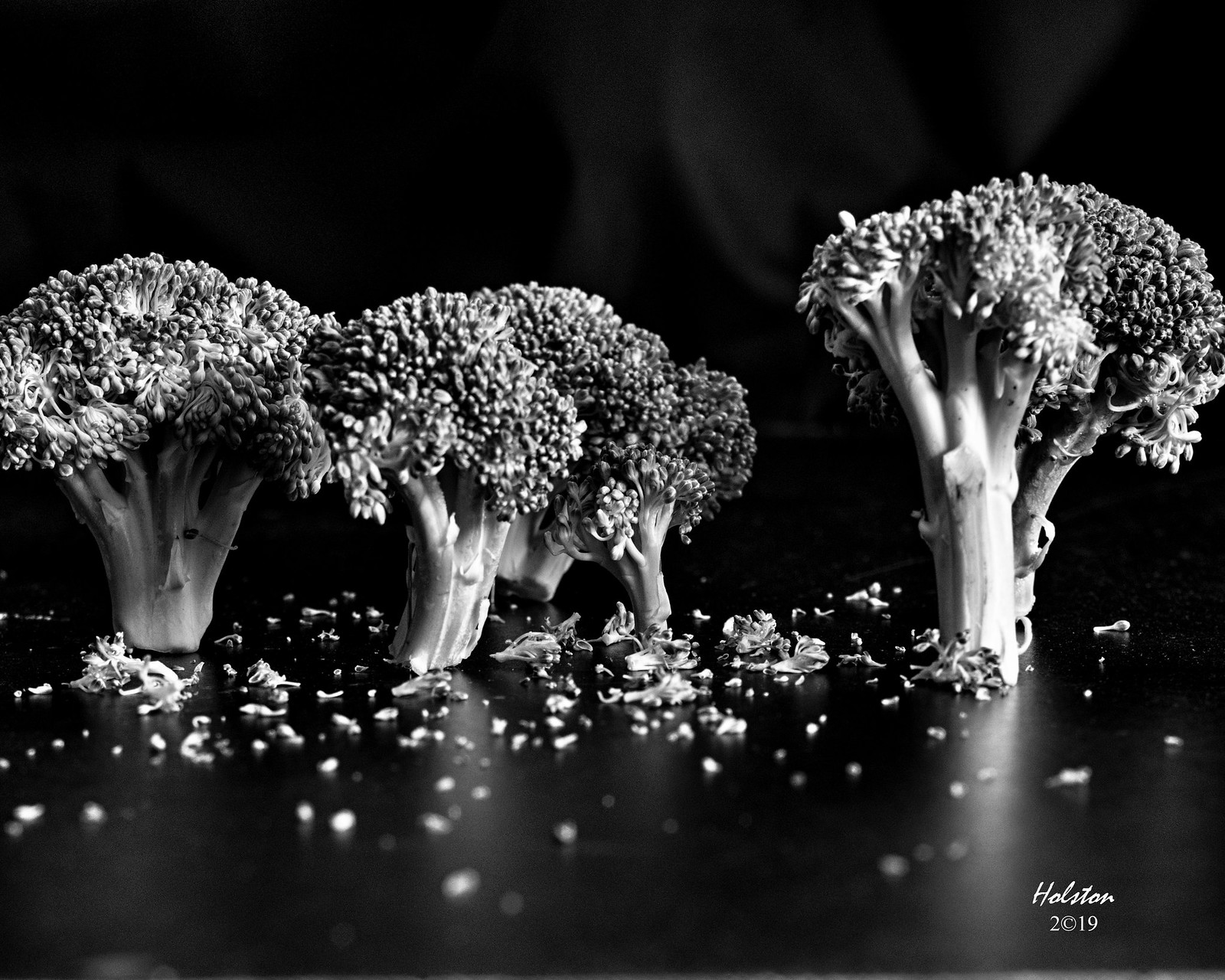This artistically professional black-and-white photograph by Holsten, captured in 2019, features an imaginative scene of four to five broccoli crowns artfully arranged to resemble trees standing upright. The high-contrast image, with deep blacks, bright whites, and a balanced middle gray range, showcases a sharp focus on the broccoli in the middle, while the foreground blurs slightly and the background is enveloped in complete darkness. The dark tabletop surface below the broccoli is sprinkled with fallen broccoli florets, mimicking leaves scattered around tree trunks. The lower portion of the image reveals reflections of the broccoli stalks, adding depth to the scene. In the lower right-hand corner, the photographer's stamp "Holsten 2019" is visible in white text, adding a professional signature to this creatively composed photograph.